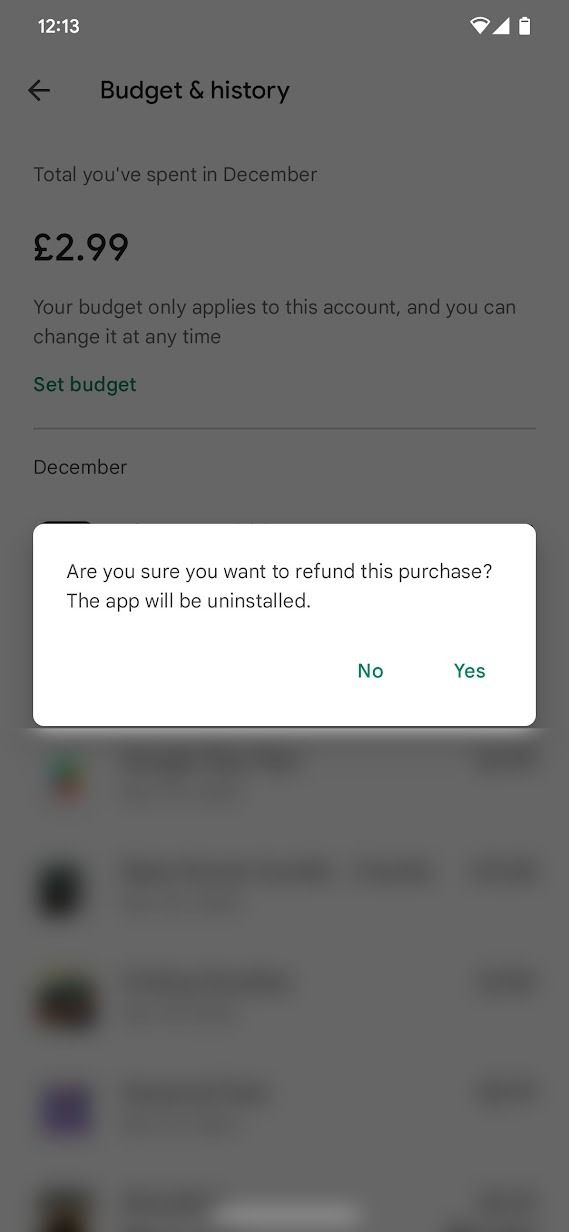The image depicts a cell phone screen displaying a financial management app. In the upper left corner, the time is shown as 12:13, while the upper right corner features icons for Wi-Fi, signal strength, and battery level. A white pop-up box dominates the foreground, asking, "Are you sure you want to refund this purchase? The app will be uninstalled." This message is accompanied by two green buttons labeled "No" and "Yes."

In the background, partially obscured by the pop-up, the app's main screen reads "Budget and History." Below this header, it shows the total expenditure for December, indicated as £2.99. There is additional text specifying that the budget applies only to the current count and can be modified at any time. A green "Set Budget" button is placed just below this message. Following a dividing line, the section labeled "September" appears, underneath which other blurred-out applications are vaguely visible.

The background of the phone screen is dark, providing contrast to the white pop-up box with its black border. The top portion of the screen is somewhat more illuminated, though still retaining a darker, subdued appearance.